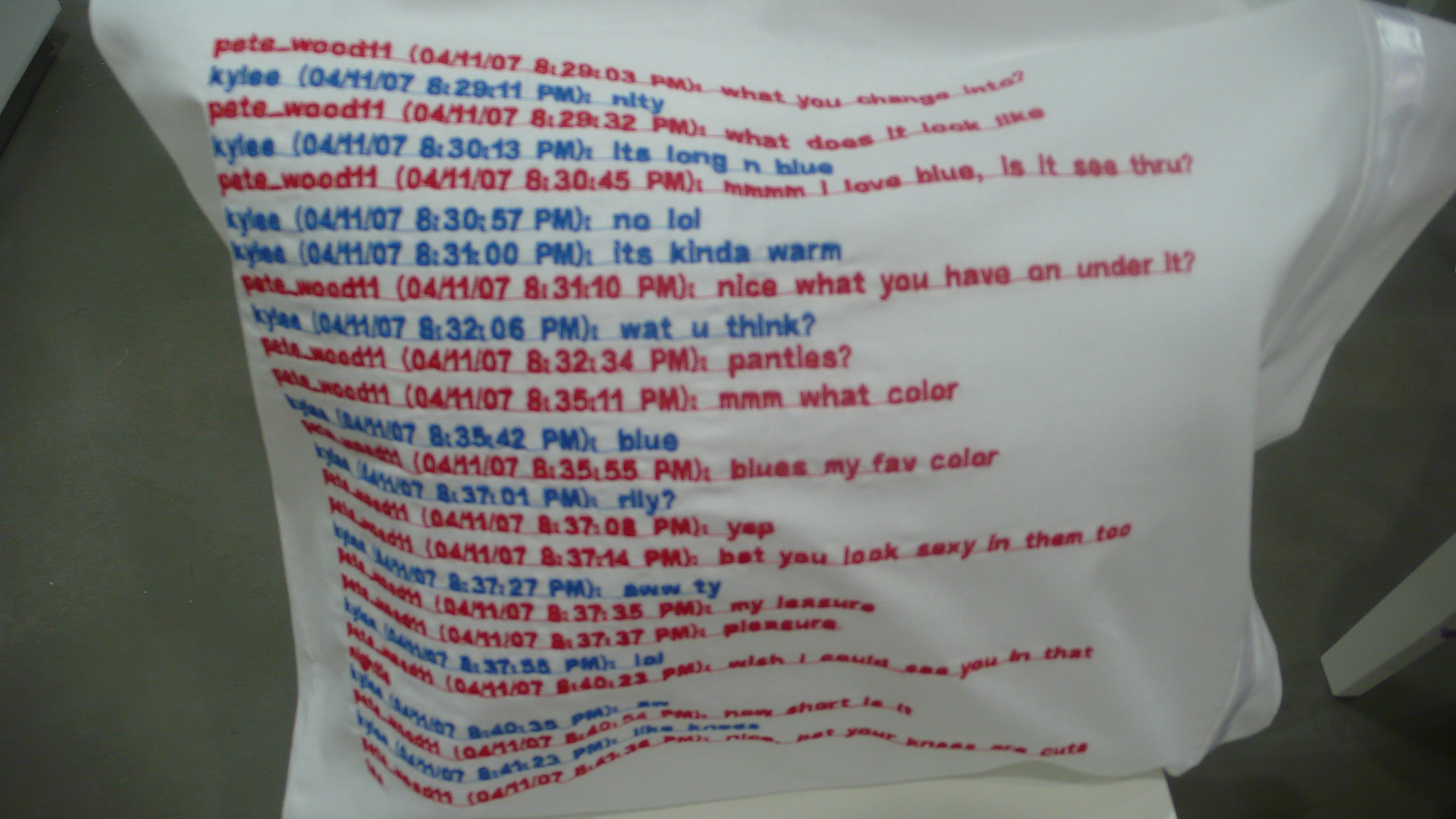The image depicts a piece of white fabric, which may be a pillowcase or similar item, draped over the back of a chair. The fabric features a printed chat log with dialogue in two colors: red and blue. The red text belongs to a user identified as Petewood11, and the blue text belongs to a user named Kylie. The conversation appears to be from 4-11-07, detailing an explicit exchange between the two participants. The timestamps for each message are precise down to the second. Notable features of the fabric include shiny edging on the right side with a more matte finish in the center and left side. In the background, a gray floor or countertop and a white chair or table leg are visible. The printed text includes various details of the chat such as questions, responses, and a few typos, reflecting an intimate dialogue. Some areas of the text are blurry and illegible, especially on the left side of the image.